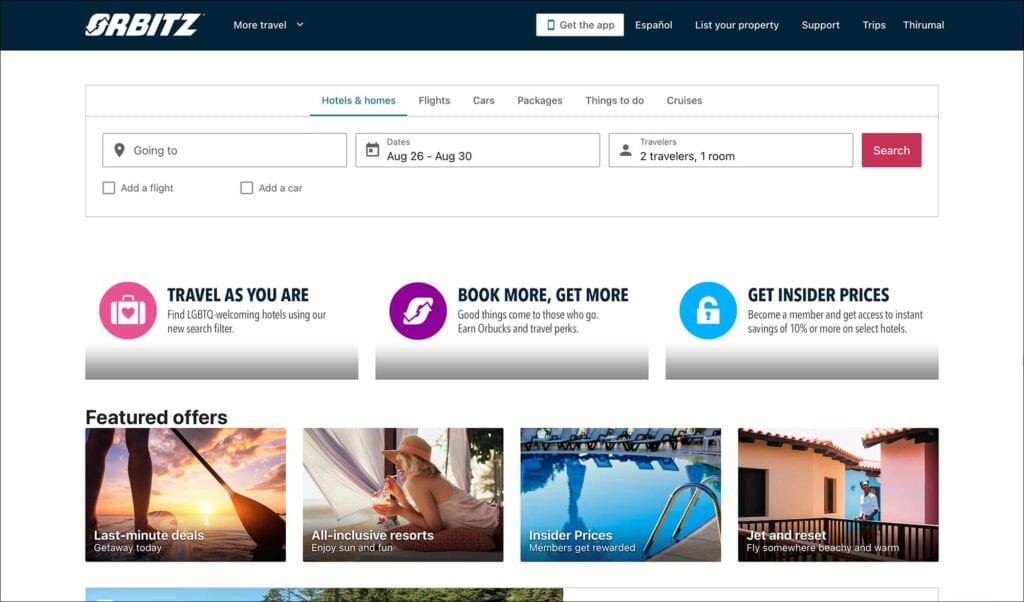The web page for Orbitz, spelled O-R-B-I-T-Z, is prominently displayed in large white letters in the top-left corner. Adjacent to it, in smaller white letters, is the phrase "More travel," accompanied by a downward-pointing arrow. This is all situated on a black banner that spans the top of the page. 

Within this black banner, several tabs are visible on the right side. The first tab, highlighted in a white box, features a green phone icon and the text "Get the app." Following this are the tabs "Español," "List your property," "Support," "Trips," and "THIRUMAL." These tabs are neatly aligned and organized for easy navigation.

Below this banner lies a white background, dominated by a large rectangular section. At the top of this section are tabs labeled "Hotels and Homes," "Flights and Cars," "Packages," "Things to Do," and "Cruises." The "Hotels and Homes" tab is highlighted in green.

Further down are three smaller rectangles. The first one reads "Going to," the second, featuring a calendar icon, shows "Dates" with the specified range of August 26th to August 30th. The third rectangle, with an icon of travelers, indicates "2 travelers, 1 room." To the right of these options is a prominent red search button with white text.

Below the search button are two checkboxes labeled "Add a flight" and "Add a car," followed by three additional rectangular boxes. The first has a luggage icon inside a pink circle and the text "Travel as you are." The second features a recycling arrow and the phrase "Book more, get more." The last one has an unlocked padlock icon with the text "Get insider prices."

Additionally, there are four images arranged below these elements:
1. A person standing on a surfboard, seen from the knees down, as they gaze at a sunset.
2. A woman lying on her stomach inside a white tent, wearing a sun hat and sunglasses while sipping a drink.
3. A house, presumably one that can be rented as part of a vacation package.
4. A scenic picture of blue water.

The layout is clean and user-friendly, designed to facilitate easy navigation and emphasize the various travel options and deals available.